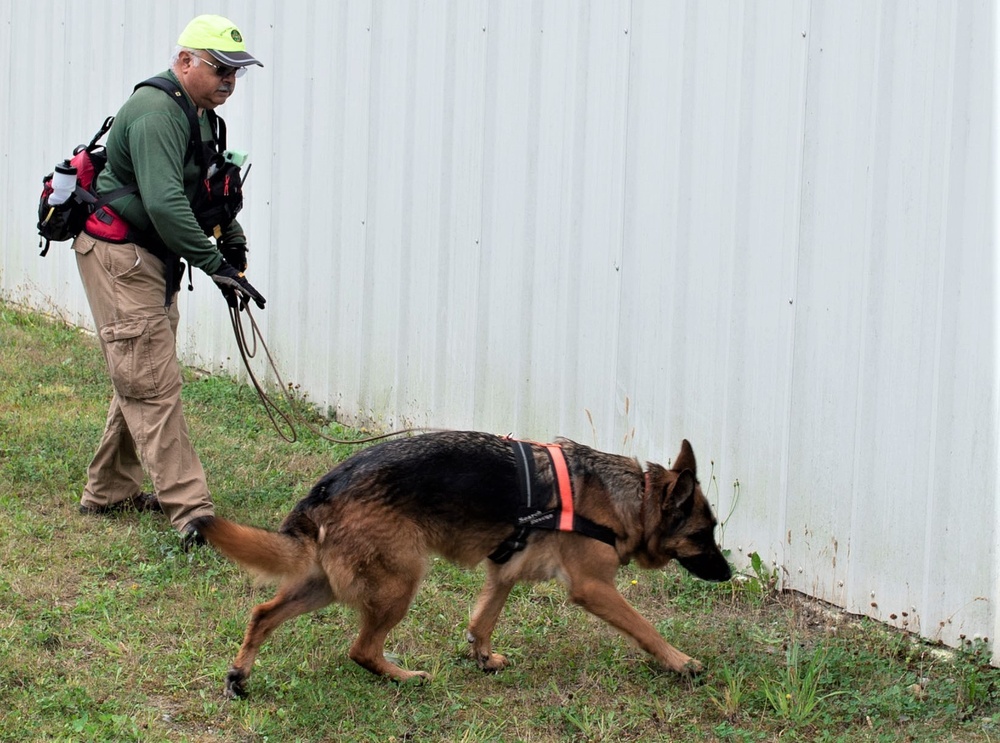The image captures a focused moment between a handler and a German Shepherd engaged in a training exercise. The scene is set in a grassy area beside a large, white wall, possibly the side of a building or a cargo crate. The German Shepherd, equipped with a black and orange harness, is sniffing the ground near the wall, appearing to search for something. The handler, an older and slightly larger man, holds the dog’s leash. He's dressed in a green long-sleeved shirt, khaki pants, and a yellow baseball cap, with tactical gear strapped to his belt and shoulders. He also carries a backpack that has a water bottle visible. The scene, likely captured during the day, shows both the trainer and the dog diligently working together in what appears to be a training scenario. The grass is green but slightly overgrown, adding to the natural, unkept setting of the image.